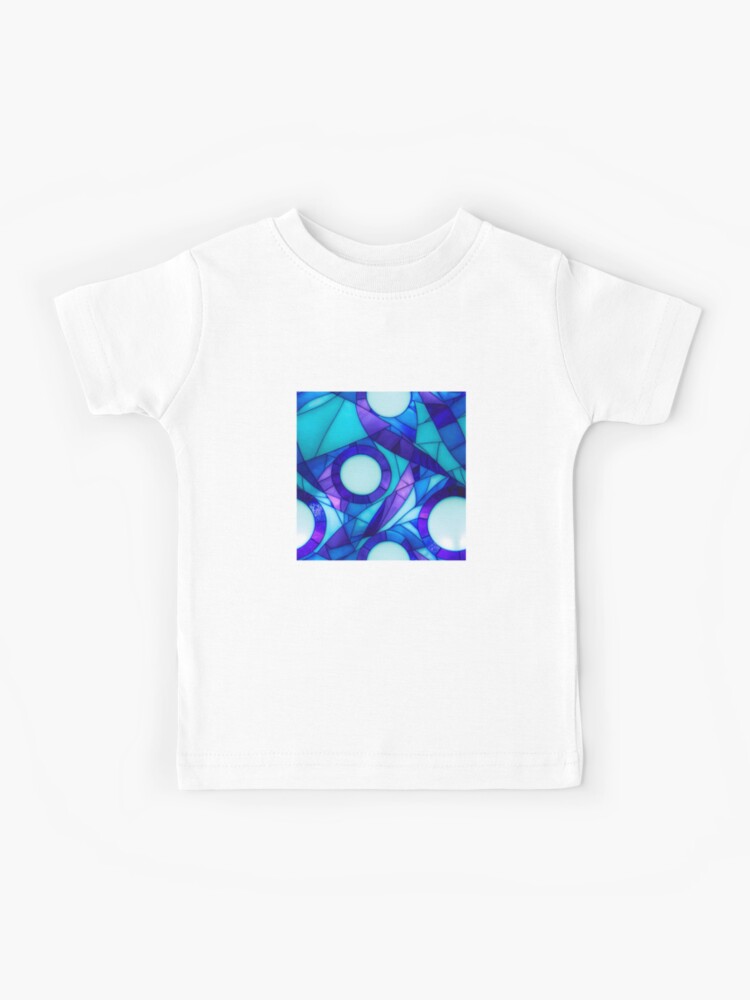This is a photograph of a pristine white, short-sleeved t-shirt lying flat against a plain white background, resembling a stock photo or one that might be used in a magazine or online retail. The focus of the image is a striking, square geometric design centered on the chest area of the t-shirt. This design is reminiscent of stained glass artwork, featuring an intricate pattern composed of various geometric shapes such as squares, triangles, and circles. The circles are predominantly light blue, with some circles outlined in dark purple and others showing gradients of dark purple to light blue. The remaining geometric shapes within the design display a palette of blue, teal, turquoise, and multiple shades of purple and green. The vivid and detailed design stands out brightly against the clean white fabric of the t-shirt, making it highly eye-catching and visually appealing.